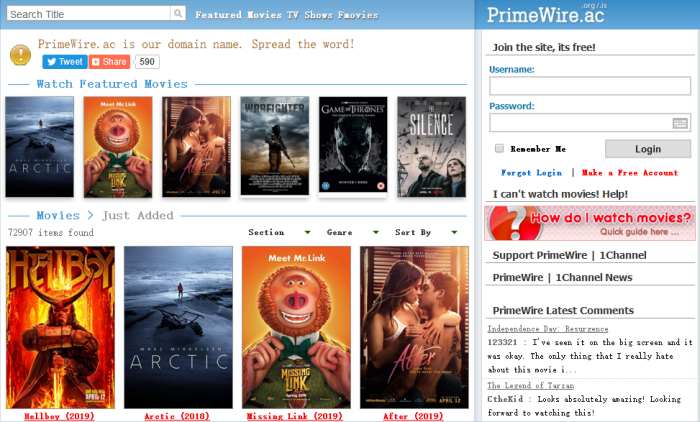This is an image of a media website dedicated to books and movies. The upper left-hand corner features a light blue banner with a long rectangular search box labeled "Search Title," accompanied by a magnifying glass icon. Towards the center, blurred text lists categories such as "Feature Movies," "TV Shows," "Favorite Movies," and possibly "F Movies." Above these categories, the domain name "primewire.ac" is displayed with the tagline "Spread the Word," alongside a caution sign, a Twitter Tweet button, and a share button, with the number "590" beneath them.

Below this section, there is a headline "Watch Featured Movies," followed by a row of six movie titles, starting with "Arctic" and ending with "Silence." Beneath this row, another section labeled "Movies Just Added" showcases four additional movie titles, including "Hellboy," "Arctic," and "Meet Mr. Link." These titles are highlighted in red font.

On the right-hand side of the page, the domain name "primewire.ac" is displayed again above a sign-in section that reads "Join the Site, It's Free." This section includes fields for "Username" and "Password," along with options for "Remember Me" and a "Login" button. Below the login area, there's a banner titled "Watch Movies," followed by further related information.